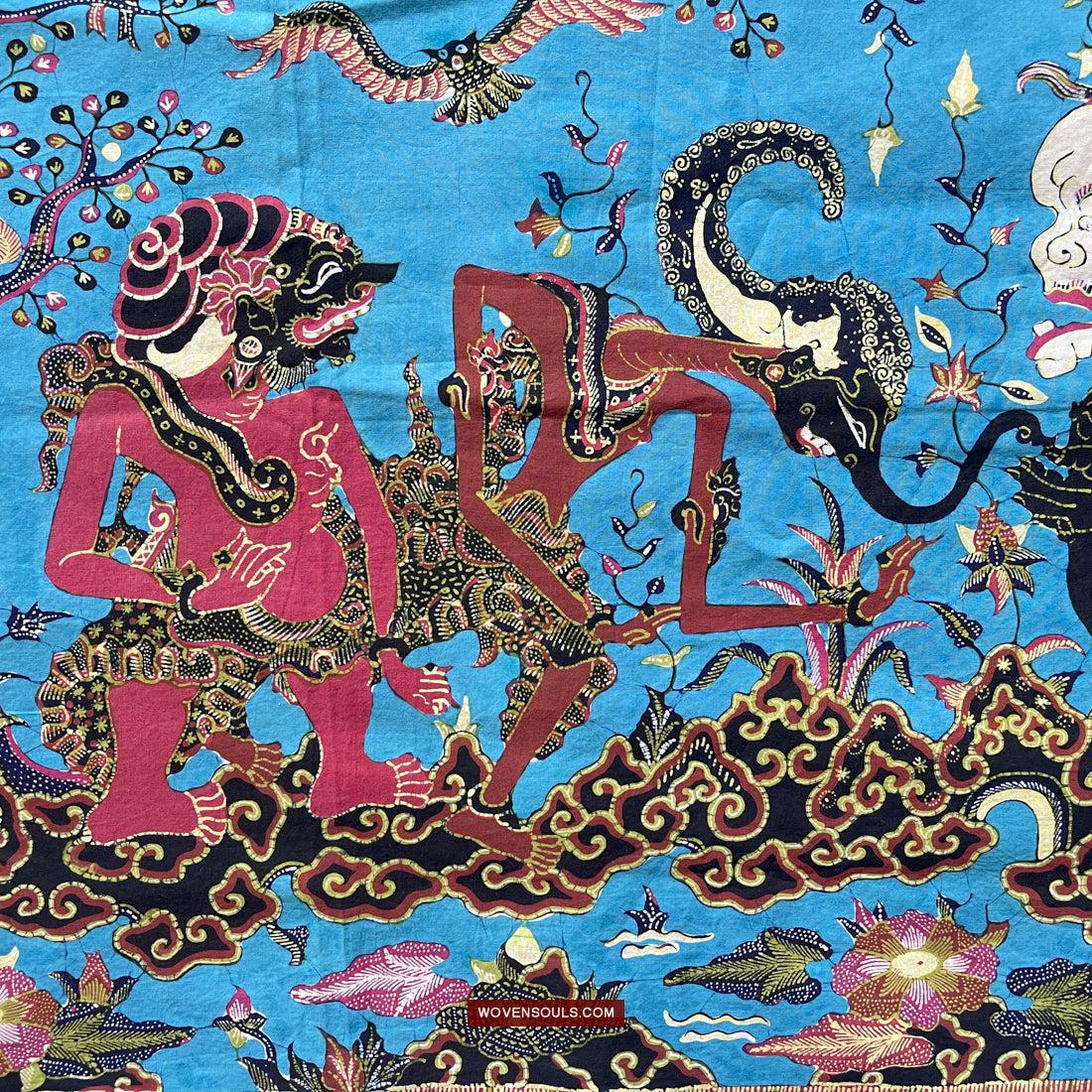This intricate tapestry from wovensouls.com primarily features a sky blue background, adorned with a vivid array of unique and surreal elements. At the bottom, a rust-colored banner prominently displays the website's name. The tapestry showcases a fantastical scene with several upright, human-like figures possessing distinctly non-human attributes. One figure, with a pink or plum body, has a somewhat disfigured face that mimics human features adorned with pink lipstick, yet its hand resembles fish fins. Another figure, with a rust-colored body, appears to combine an elephant's trunk with an octopus tentacle emerging from its head. An additional figure has a black body, contributing to the tapestry's eclectic palette.

Above these figures, an oddly shaped bird soars, adding to the tapestry’s surreal quality. They are depicted walking on a path that features intricate paisley patterns blending rust and black hues. Surrounding the figures, the scene teems with nature-inspired designs, including non-realistic, vibrant trees, and plants, along with what appear to be pink lily pads and various animals, including an owl. The entire composition is rich in diversity with a complex interplay of different shapes, designs, and a myriad of colors, creating a lively and imaginative tableau with potential religious or mythological undertones.